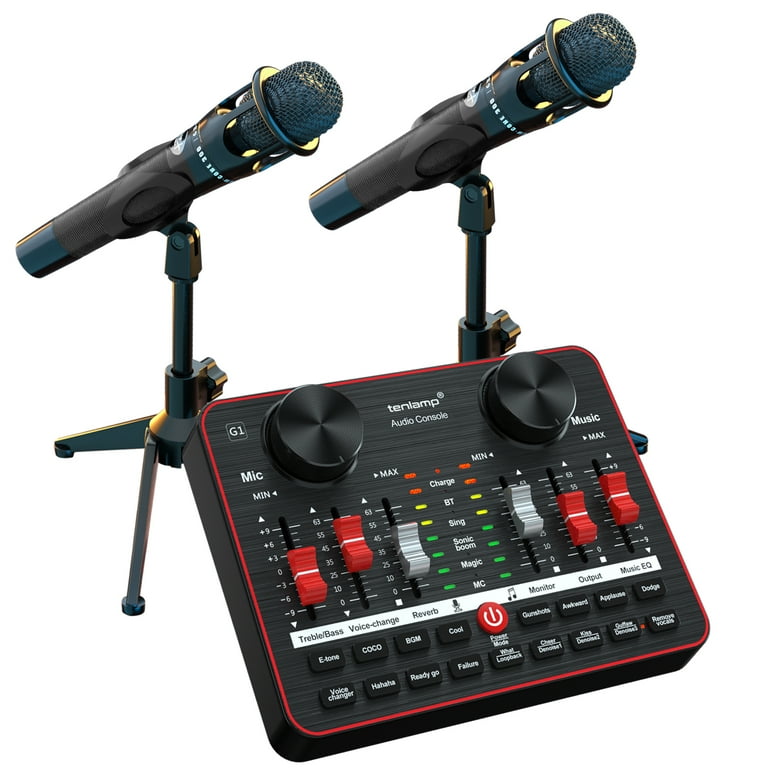The photograph showcases a black 10-lamp audio console set against a completely white background. This professional recording equipment features an array of red and white slide buttons and multiple small, labeled buttons whose text is unreadable. Dominating the front of the console are two distinctive knobs—one labeled 'mic' and the other 'music', both marked with 'min' and 'max'. There are three red and three white sliders on the left side under 'mic' and on the right side under 'music'. In the center of the console is a conspicuous red power button, surrounded by about 16 or 17 smaller buttons in two rows. The edges of the console are accentuated with a strip of red paint. Additionally, the equipment includes two black microphones with blue accents, mounted on black and blue adjustable stands positioned behind the console. The microphones appear to be integrated into the setup, adding to the professional aesthetic of the image. Various switches and labels such as treble, voice change, and music EQ are also visible on the device, enhancing its functionality and complexity.